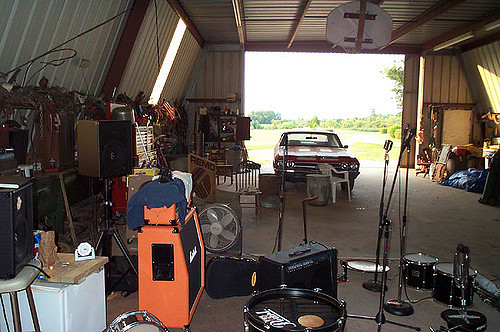The photograph captures the interior of a very large, tan-colored garage or pole barn, characterized by brown supports on the ceiling and sidewalls, and metal panels lining the interior. The open overhead door reveals a bright, sunny day with a tree line in the background. Dominating the scene is an antique red muscle car, distinguished by two white racing stripes on the front and visible headlights, parked towards the back. 

The spacious interior is cluttered with various items, suggesting an eclectic mix of storage and use. Prominently featured is a collection of music equipment including an orange amplifier, a black amplifier, numerous speakers, microphones, and various parts of a drum set. There are also practical utility items scattered around, such as a toolbox, box fans, and miscellaneous boxes likely filled with tools or other general items. Additionally, a basketball hoop is mounted on the ceiling, further emphasizing the multi-functional nature of this expansive garage.